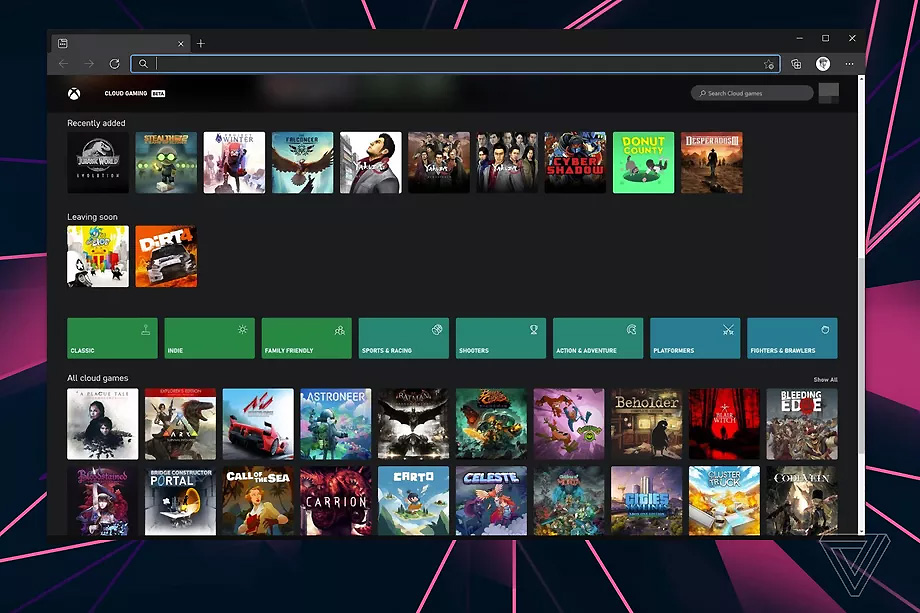Screenshot of a Web Page: 

The image displays a screenshot of a webpage primarily with a dark background peppered with accents of pink, burgundy, and purple lines interspersed with white spaces. At the top of the page, there is an empty search bar outlined by a vivid blue border, contrasting against its black interior. In the upper-right corner, the Xbox symbol is visible along with text indicating “Cloud Gaming” followed by a “Beta” label housed in a white rectangle.

Down the left-hand side of the display, a section labeled “Recently Added” lists several games, though some titles are partially obscured. Visible titles include "Jurassic World," "Stealthics," and a game with the word "winter" in its title, featuring an eagle on the cover. Other partially visible titles appear to be "Yankee," "Yozam" (twice), followed by "Cyber Shadow," "Donut County" (or "Country"), and "Desperados."

Further down, the “Leaving Soon” section showcases two highlighted games, one of which is labeled "Dirt." Below this, various categories such as “Classic,” “Family-Friendly,” “Indie,” and other genres are listed, leading to a section at the bottom titled “All Cloud Games,” displaying numerous game cover images organized within their respective categories.